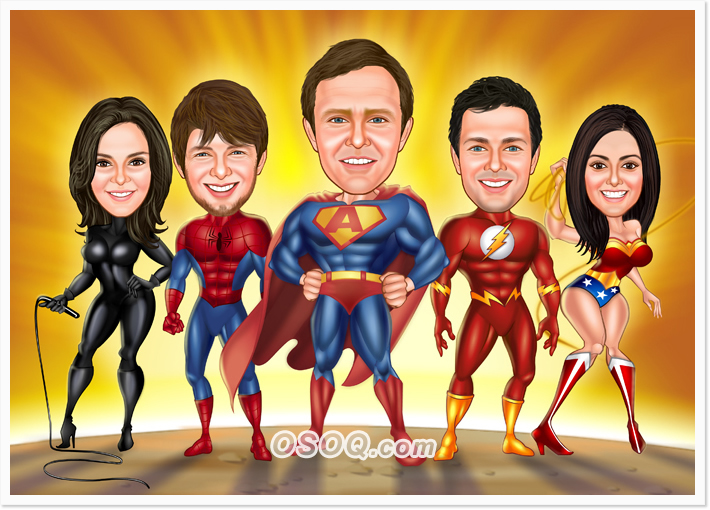The cartoon illustration showcases a lineup of famous superheroes with exaggerated human faces superimposed onto their bodies, all standing on a beige stage with a radiant gold and orange background. Starting from the far left, the first character is a rendition of Catwoman, dressed in a tight black unitard that accentuates her curves, holding a black whip at her side. Her face, an oversized drawing of a Caucasian woman with long dark hair and pinkish facial features, is disproportionately large for her body. Next is Spider-Man in a blue chest unitard with red gloves, boots, and a partial beard. His human face, also enlarged, depicts a smiling young man with tousled brown hair. The center figure appears as a Superman-like character with a unique 'A' insignia on his chest instead of the traditional 'S.' He dons a blue suit, red trunks with a yellow belt, red boots, and a cape. The face, oversized and possibly middle-aged, features fair skin and brown hair. To his right stands a character resembling The Flash, outfitted in a red suit with yellow boots and a prominent lightning bolt design. The face here is again disproportionate, showing a young man with dark brown hair. The final character on the far right is Wonder Woman, wearing a red and gold bustier, blue trunks with white stars, and red knee-high boots. She holds a string above her head, and her oversized face shows a young woman with long, dark brown hair flowing past her shoulders. At the bottom of the image is a superimposed website address: "osoq.com." This colorful and vivid depiction merges superhero iconography with cartoon-style human facial features.